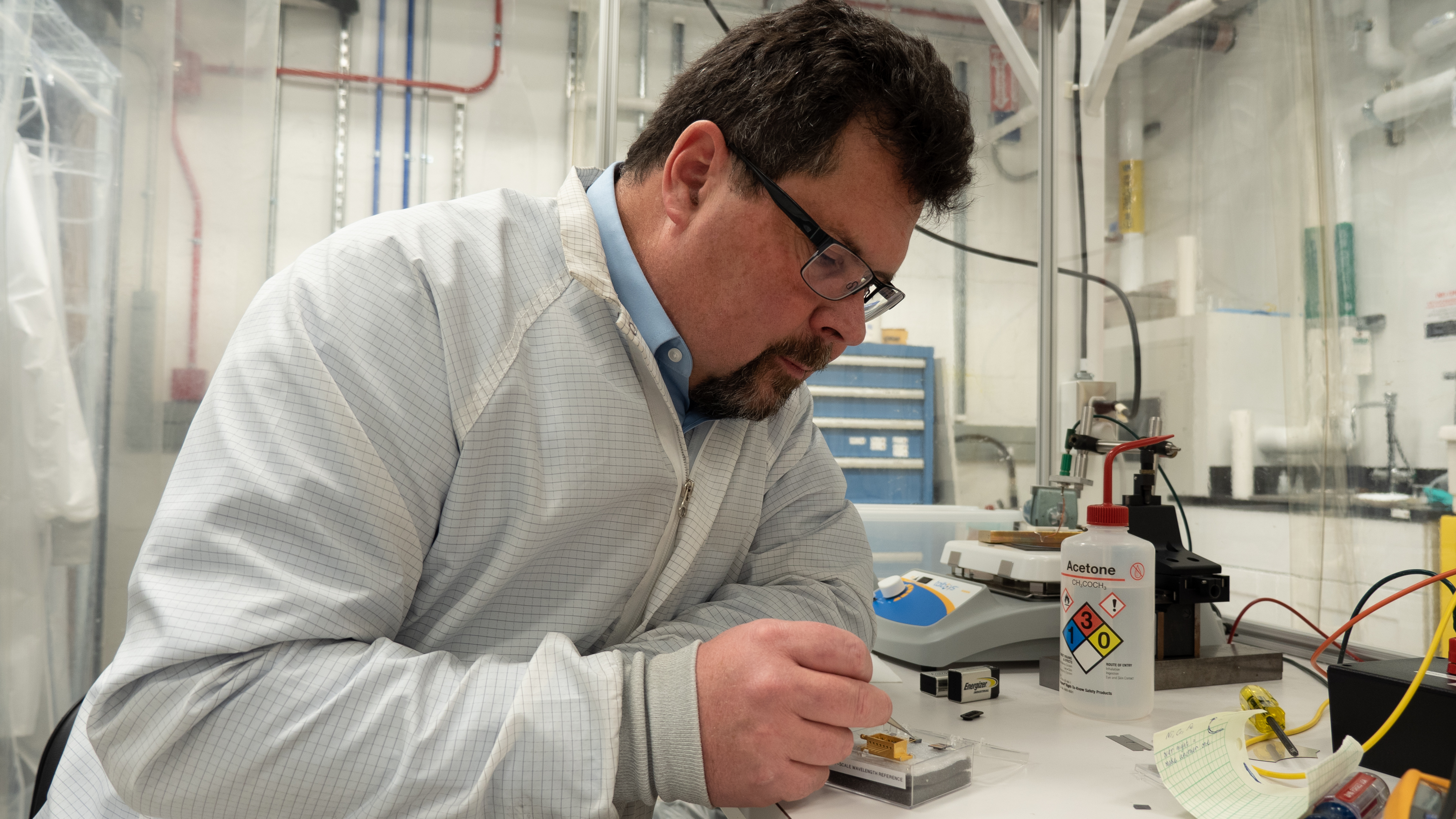In this detailed, full-color horizontal photograph taken indoors under artificial light, a scientist is seen meticulously working in a predominantly white laboratory, characterized by its white walls and an array of white pipes carrying various gases and liquids. The scientist, captured in profile in the center of the image, has short, curly dark hair and is wearing black glasses along with a brown goatee. Dressed in a blue button-up shirt beneath a white sanitary jumpsuit, he is focused on his task at hand.

The scientist is engaged in some intricate work involving machinery and wires at a desk or table, using what appears to be a pair of tweezers. A variety of testing equipment and wires are spread out on the table behind him, further emphasizing the lab setting. A notable object in the scene is a plastic squeeze bottle on the desk, adorned with a diamond-shaped label featuring colors white, blue, red, and yellow, likely indicating the chemical contents within. The overall palette of the image includes additional tones such as off-white, light blue, teal green, and black, contributing to the sterile yet scientific ambiance of the laboratory space.